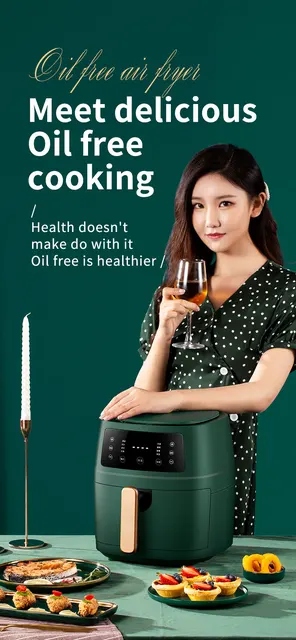The advertisement showcases a sophisticated and elegant scene featuring an oil-free air fryer. Set against a predominantly dark green background, the ad begins with the gracefully scrolled text "Oil-Free Air Fryer" in pale yellow. Just below, in a bold, chunky white font, it reads, "Meet delicious oil-free cooking." Further down, in a smaller, white font, it continues, "Health doesn't make do without it. Oil-free is healthier."

At the center of the image is a young Asian woman with her long hair partially clipped back above her left ear with a white clip. She is elegantly dressed in a dark green dress adorned with white polka dots and two large white buttons. In her right hand, she holds a glass of white wine, while her left arm rests casually on top of a sizeable dark green air fryer with a pale gold handle.

The air fryer stands on a pale green table, which is adorned with an array of colorful and delectable dishes. These include fruit tarts, fish, peppers, meatballs, and various other vibrantly colored meals. A single white candle in a candle stand and a white and pink cloth under one of the dishes adds to the charm and elegance of the setting.

The visual appeal and detailed presentation effectively highlight the benefits and sophistication of oil-free cooking, making a compelling case for a healthier lifestyle.